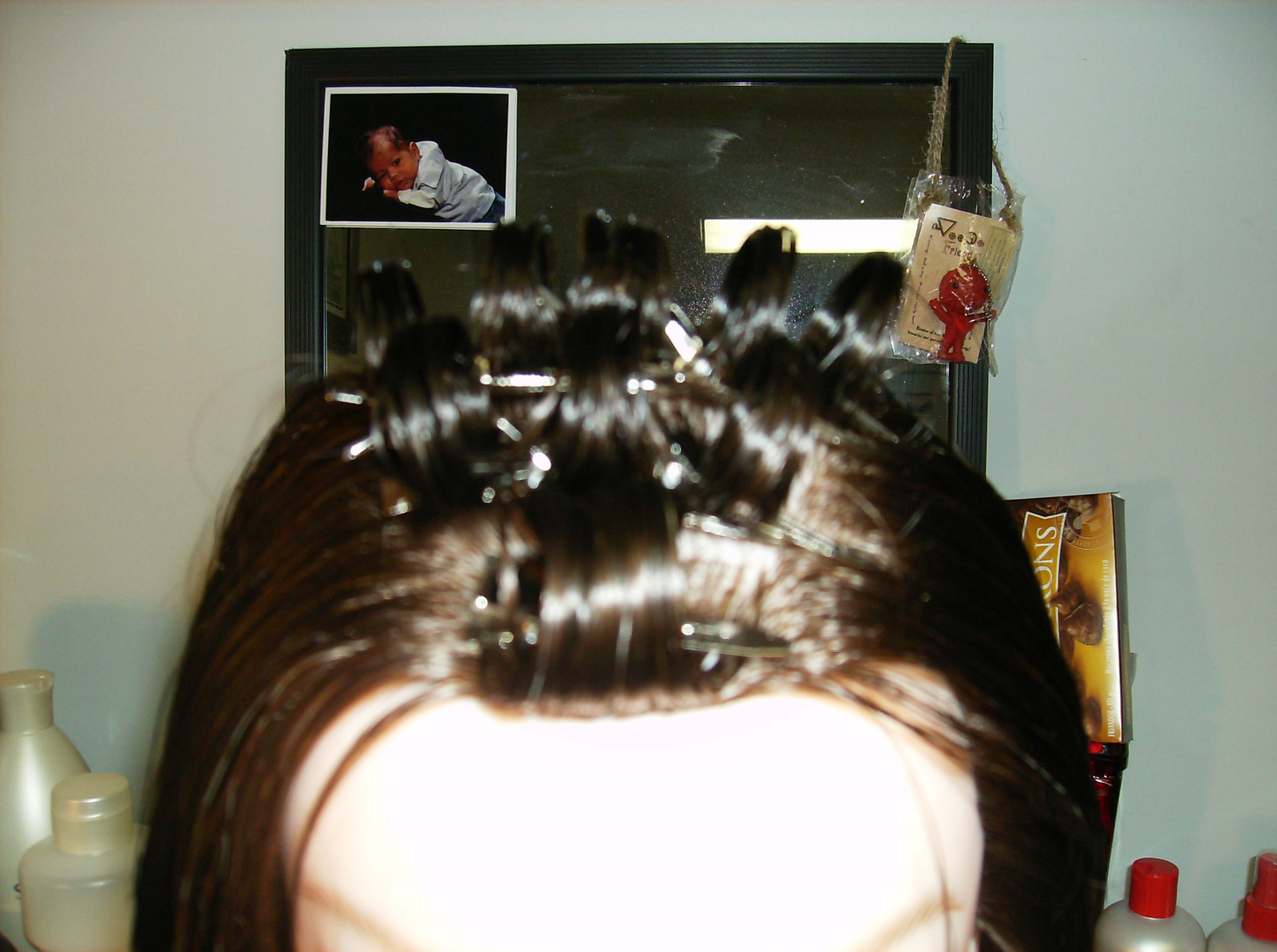The image captures a close-up shot of the top of someone's head, specifically showcasing a dark brown hairstyle. The top and bang section of the hair is intricately styled into tight curls or rolls, secured with numerous silver barrettes and hairpins, giving a detailed look at the pinned-back design. The hair on the sides flows straight down, contrasting the elaborately styled top. The background features a mirror outlined in black, with a baby’s photo affixed to its upper left corner. Next to the baby’s picture is a small red plush toy encased in a plastic container, suspended by a string. Below the mirror, several bottles are visible on a counter — two white bottles on the left, and two more with distinct red lids on the right. The wall behind these items is a whitish-gray, adding a neutral backdrop to the scene.